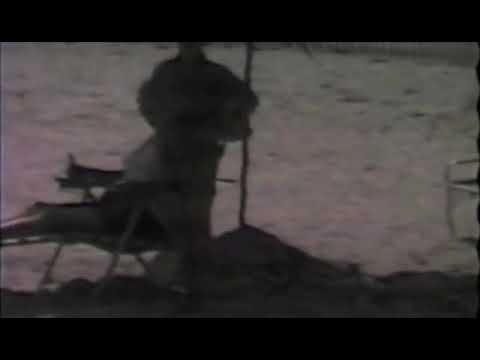The image depicts a low-resolution, black-and-white outdoor scene that appears to be on a beach, dominated by various shades of gray and brown. In the left half of the image, a person is sitting in a beach or lawn chair, with their legs reclined out in front of them towards the left edge of the frame. The individual may be wearing a large hat, although it is difficult to discern due to the image quality. Standing behind and slightly to the right of this person is another figure, silhouetted in darkness, making any details indiscernible. In the background, the textured ground resembles sand scattered with debris, enhancing the beach setting. A straight pole, likely part of an umbrella, rises from the ground to the left of the standing figure, casting a shadow that darkens the foreground terrain more than the background. To the right side of the image, a portion of another beach chair is visible, suggesting more people might be present in this obscure, hazy scene.